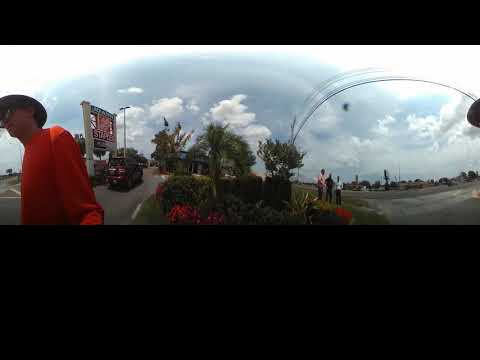The image depicts a lively entrance to a strip mall, typical of suburban America, under a clear blue sky with puffy white clouds. Dominating the left side, a man stands wearing an orange shirt, a broad-brimmed hat, and sunglasses, near a two-pillared signboard that prominently features the Staples logo, alongside other indistinct store names. Adjacent to the sign stands a parked red SUV. In the center of the scene, a green area flourishes with various trees and shrubs adorned with red flowers, indicating a possible tropical location. On the far right, three men—one in a pink top, another in black, and the third in white—engage in conversation either on the edge of the parking lot or a roadway. Adding a touch of modernity, a curved black line arches across the sky, contributing to the dynamic nature of the scenery.